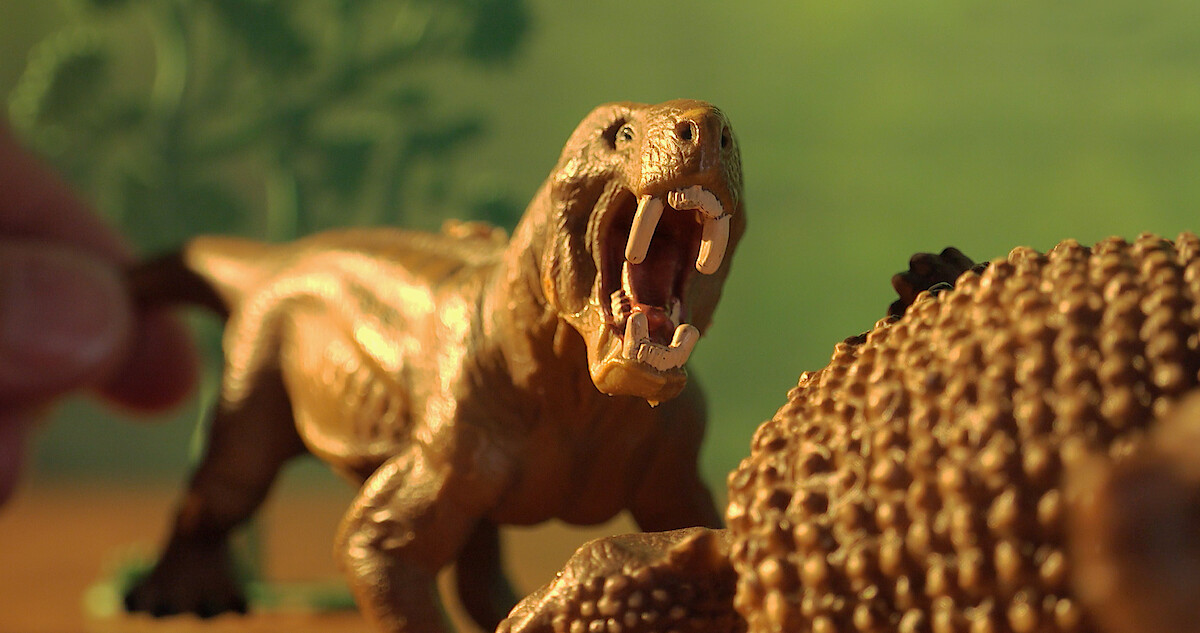The photograph captures an imaginative scene featuring toy dinosaurs, presumably set indoors with a backdrop of green plants, giving an impression of greenery. The primary focus of the image is a small, golden-brown plastic dinosaur positioned in the center. This dinosaur, possibly a T-Rex, is depicted with its mouth wide open, displaying prominent, although somewhat rounded, white teeth. A hand, slightly blurred, is visible on the left side of the picture, using fingers to hold up the dinosaur’s tail, enhancing the overall dramatic effect. To the right, partially out of focus, there appears to be another toy, perhaps another dinosaur or reptile, characterized by a spiky, scaly texture. The scene is set on what looks like a wooden table or platform, creating a miniature, yet vivid prehistoric tableau.